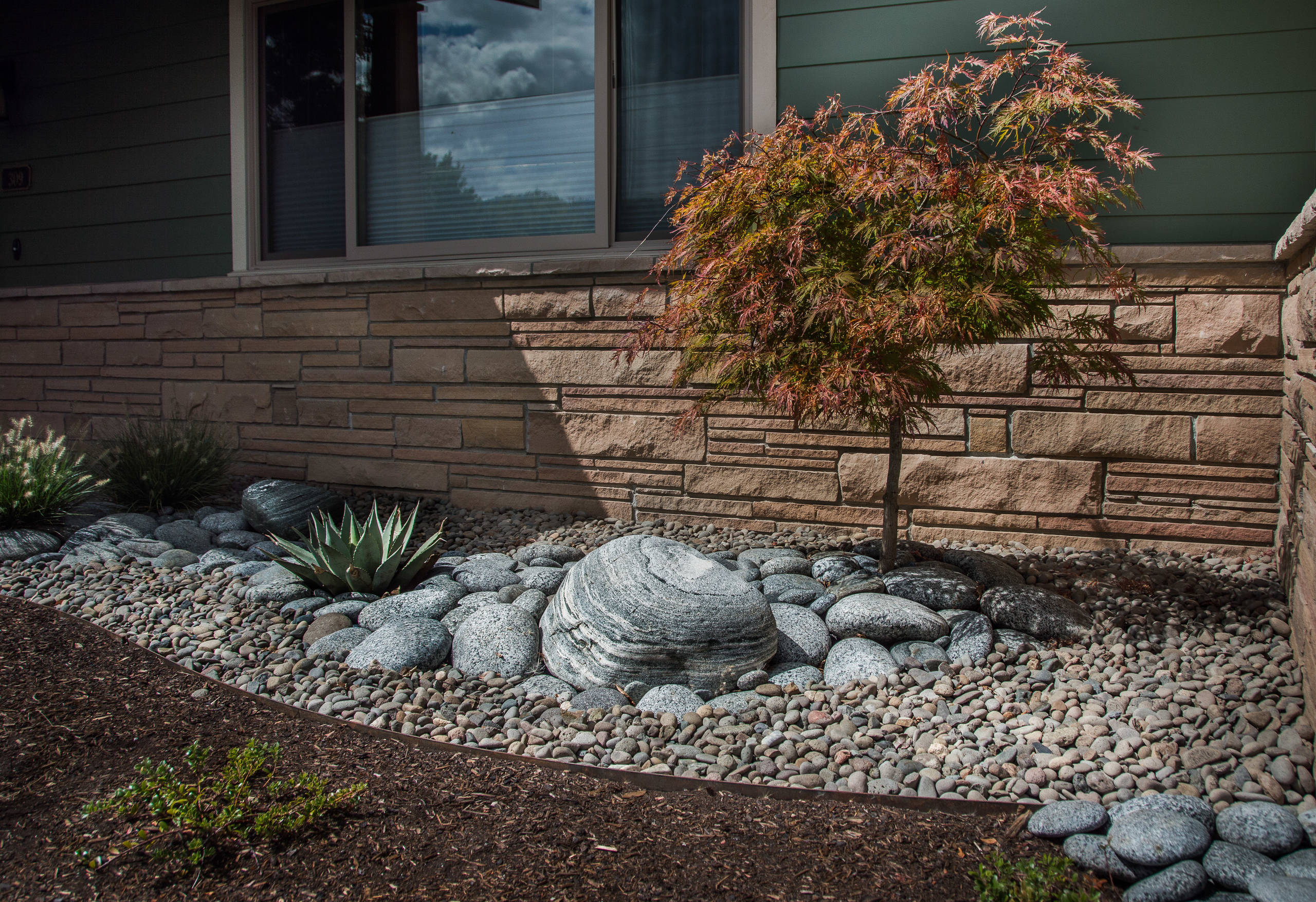This is a detailed photograph depicting the landscaping in front of a brick and siding residential house. The focal point is the intricately landscaped area adjacent to the house's foundation. The foundation is composed of light brown bricks, with a contrasting dark green horizontal plank siding above, partially visible in the background. Central to the landscaping, a river rock bed features a mix of small rocks and larger boulders arranged decoratively. 

At the base of this rock bed, there is a segment of bark mulch flanked by short, sparse grass intermingled with occasional weeds. Various plants populate the area, including low-growing ground cover and some ornamental grasses to the left. A striking succulent, likely an agave, is positioned centrally, while a small decorative maple tree with fine, variegated green to red leaves stands to the right, near the brick foundation.

In the backdrop, behind the tree, a window with blinds partially drawn reflects the daytime sky, adding a touch of realism to the scene. The landscaping design serves as both a visual and functional border, delineating the house from the adjacent grass and dirt. This photorealistic image is devoid of any text, focusing solely on the aesthetic and natural elements of the house's exterior.